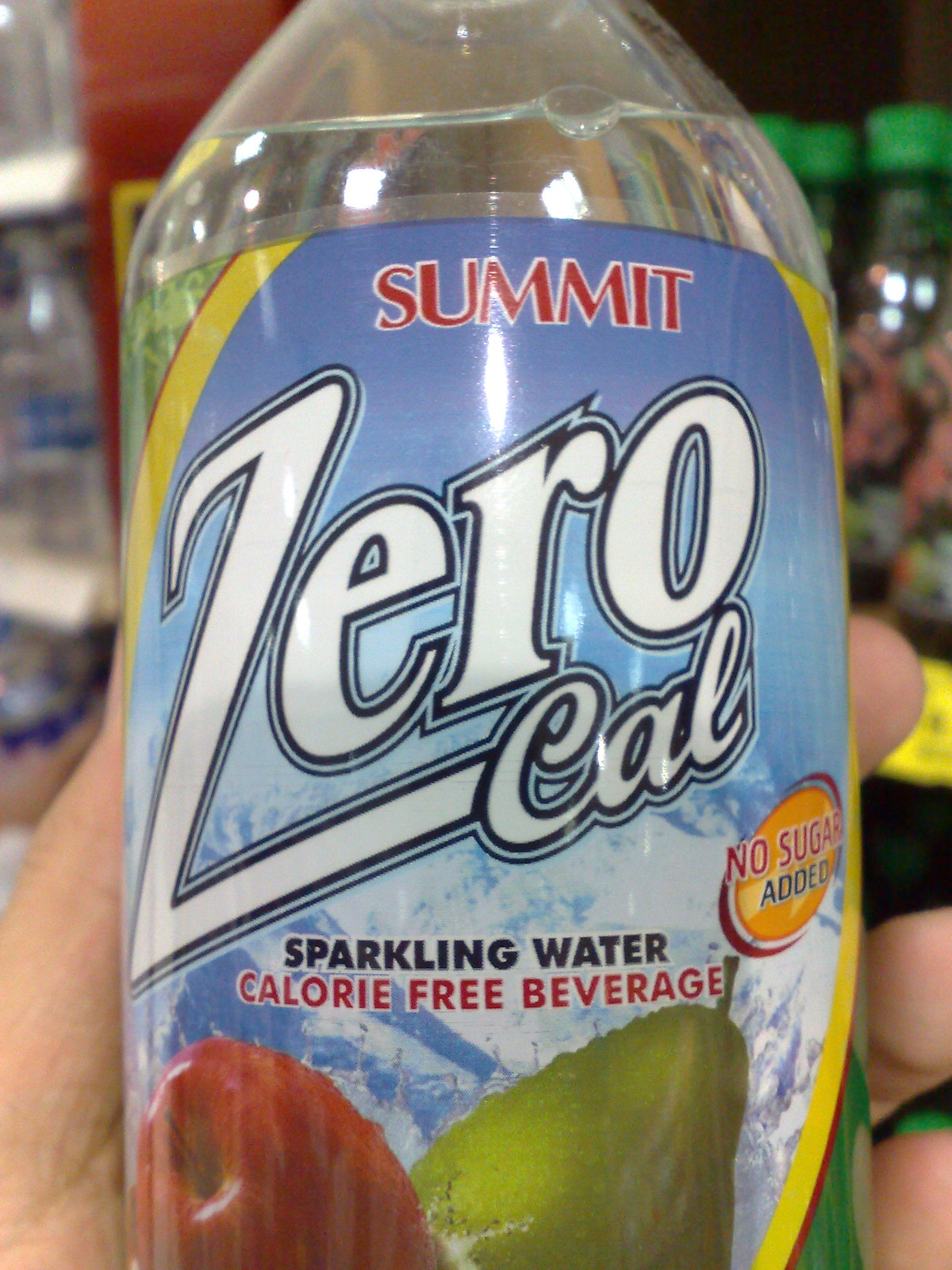In the photograph, a hand prominently displays a bottle of sparkling water labeled "Summit." The liquid inside the bottle is crystal clear, while its label is a light blue backdrop adorned with accents of yellow and green. The front of the label features images of an apple and a pear, and the text, written in white, red, and blue, reads "Summit, zero-cal, sparkling water, calorie-free beverage, no sugar added." The setting appears to be a grocery store, as evidenced by the shelving units and an array of other beverages visible in the background, including iced tea and bottled water. The composition of the image ensures that the focus is primarily on the bottle, with no other people or additional text present in the frame.